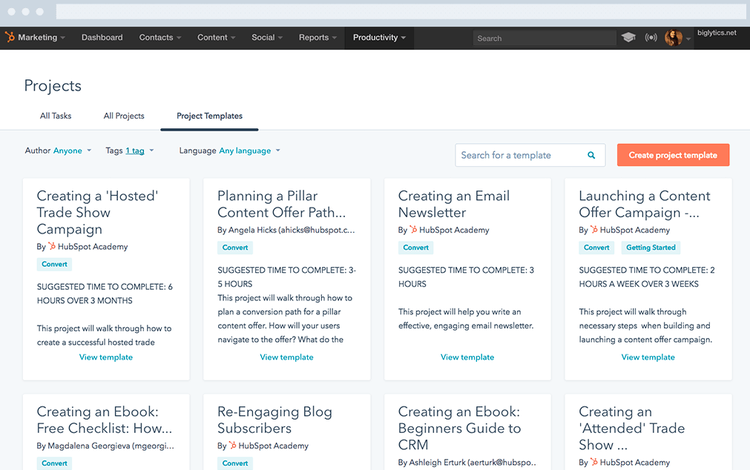The image depicts a webpage dedicated to project planning resources, specifically catering to marketing professionals. The main heading at the top of the page reads "Marketing," indicating the general focus of the content. The provider of this page, however, isn't specified. Under the prominent header "Projects," there are three subheadings: "All Tasks," "All Projects," and "Project Templates," with the latter being the selected view.

The page is organized into four main columns, each featuring a detailed description of various project templates available for use. These columns are titled “Creating a Hosted Trade Show Campaign,” “Planning a Pillar Content Offer Path,” “Creating an Email Newsletter,” and “Launching a Content Offer Campaign.” Additional templates listed include "Creating an Ebook Free Checklist," "Re-engaging Blog Subscribers," "Creating an Ebook Beginner's Guide to CRM," and "Creating Attended Trade Shows." Each template presumably provides structured guidance, steps, and necessary information to assist users in executing these marketing initiatives effectively.